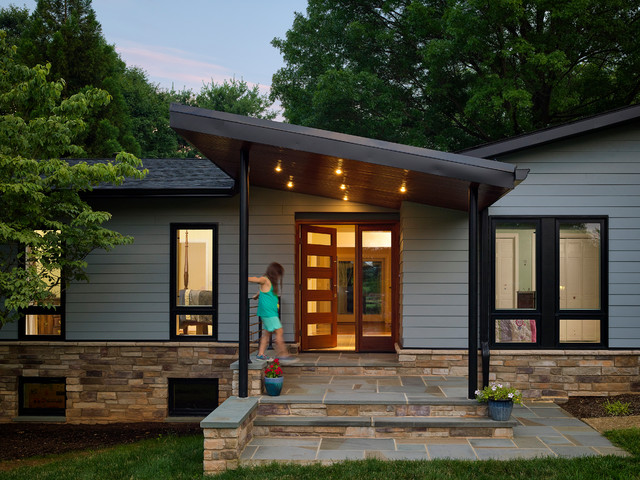The image depicts a modern gray house with black trim, featuring a combination of vinyl siding and a basement finished in rock or flagstone. A large oak tree and additional greenery frame the house against a backdrop of a clear blue sky. Centered in the image is the covered front porch, which has a slanted roof supported by black poles. The porch has three steps, with a blue flower pot containing white flowers on the second step, and another blue pot with red flowers on the porch itself. The front door, slightly ajar, is flanked by four windows, offering a glimpse into the house's interior where white closet doors and a blue-striped sofa can be seen. A young white girl, dressed in a teal tank top, teal shorts, and blue shoes, stands on the porch. The entrance, adorned with potted plants, appears both inviting and well-maintained.